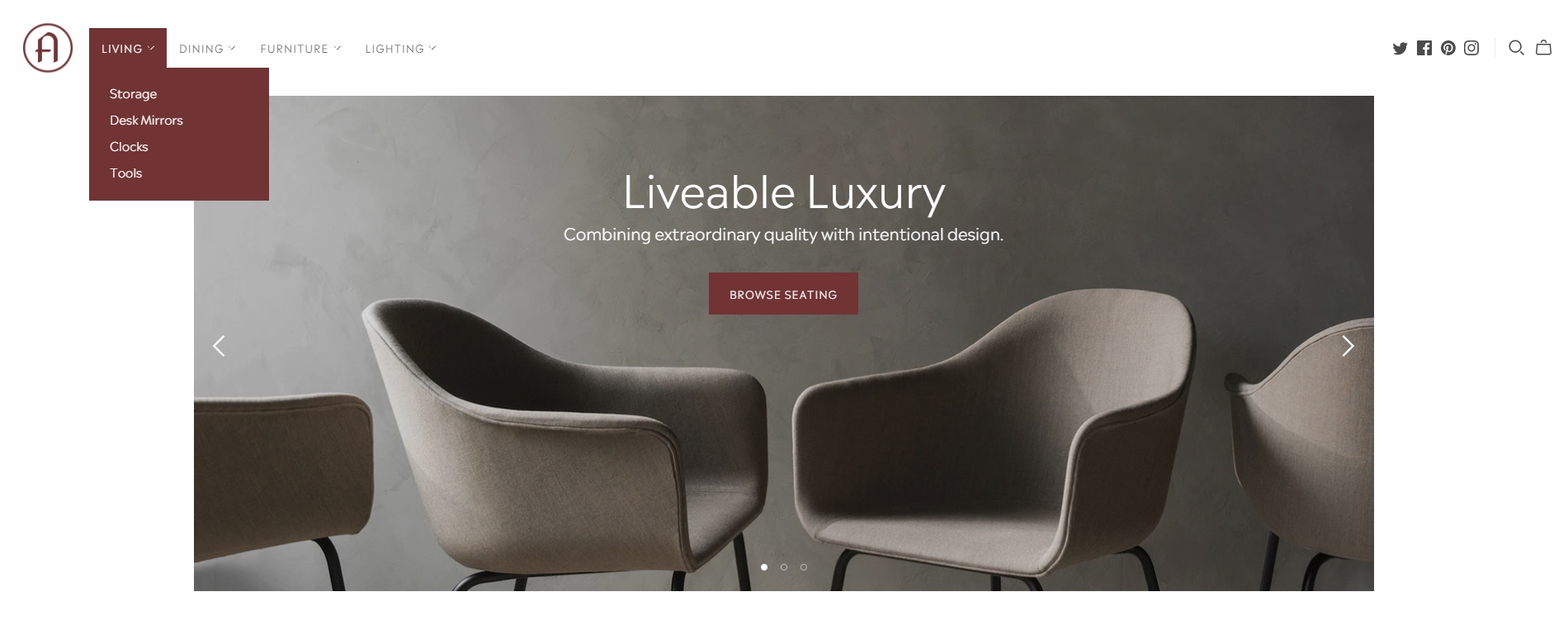The image shows a webpage with a predominantly white background at the top, featuring a red-outlined circle enclosing a red letter "A." The first tab, labeled "Living," is highlighted with a white background, while the main background of this section is burgundy. The text within the burgundy box lists categories in white: "Storage," "Desks," "Mirrors," "Clocks," and "Tools." Adjacent tabs in gray display categories like "Dining" and "Furniture."

On the right side of the header, there are various social media icons in gray: a bird for Twitter, logos for Facebook, Pinterest, and Instagram, a magnifying glass for search, and an outlined shopping bag for the cart. The main background of the picture features varying shades of gray, transitioning from lighter to darker as it stretches across the page.

In the central part of the page, bold white text reads "Livable Luxury," with a subtitle below that says, "Combine extraordinary quality with intentional design." This text is enclosed in a large, rectangular white box. Below the text are two gray chairs facing each other, and at the bottom of this section are three circles indicating pagination for a slideshow. The first circle is solid white, signaling the current slide, while the next two circles are outlined in white and transparent in the middle, indicating other slides not currently viewed.